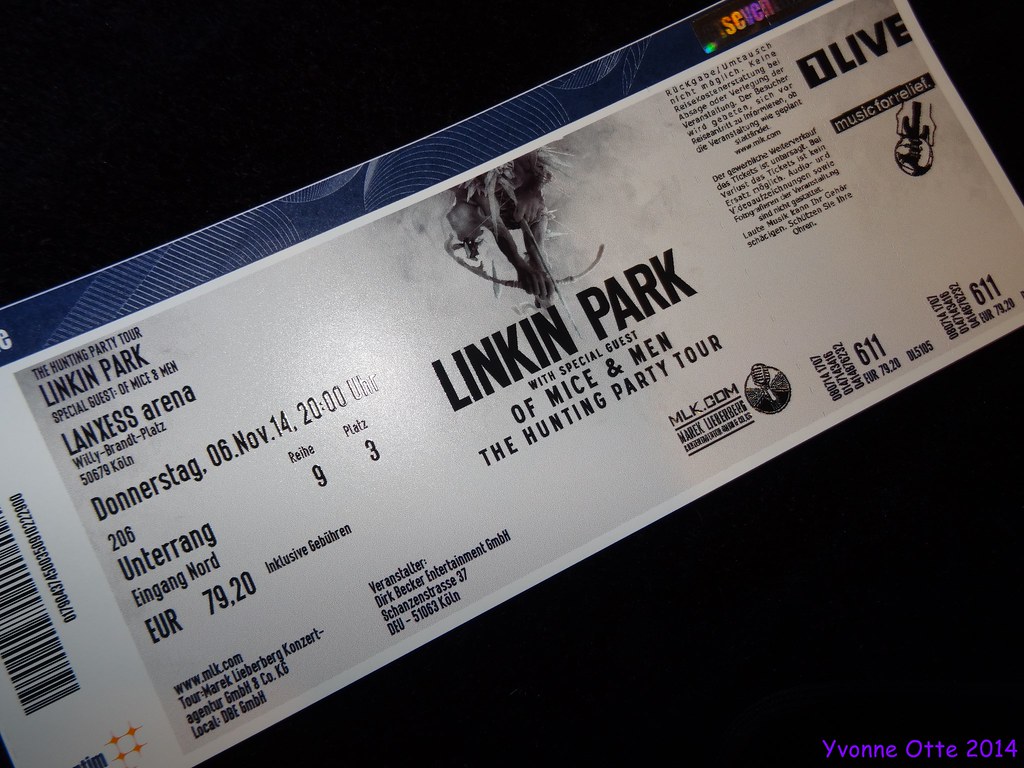The image shows an event ticket for the "Linkin Park Hunting Party Tour" featuring special guests "Of Mice and Men," set against a black background with a purple bottom right corner. The ticket, primarily in black and white with some blue at the top, indicates the event is taking place at LanXess Arena on Thursday, November 6, 2014. It includes the price of 79.20 euros. There is a barcode on the left side and a guitar image on the right. The ticket also mentions sponsors, notably One Live, and lists an address, Schanzenstrasse 37. The name Yvonne and the term "A-T-O-T-T-E" 2014 are noted, alongside other registration codes like 611 and FDRFOR79.20. Additionally, the ticket features the business name Dirk Becker Entertainment GMBH, suggesting a German origin through terms such as "Donnerstag" (Thursday) and the currency in euros.